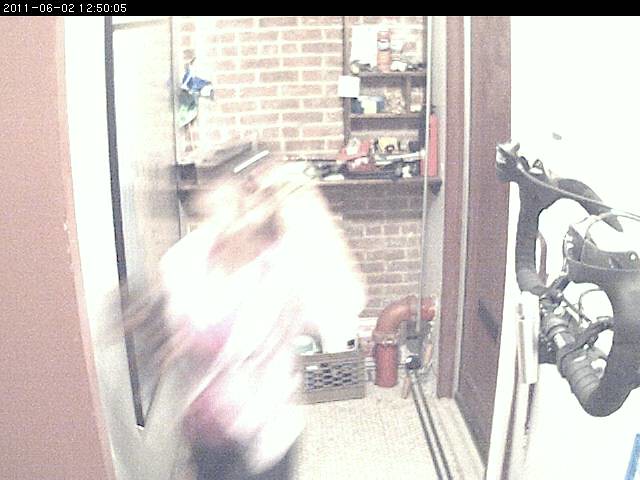An overexposed and grainy image, marked with a date stamp in a black rectangular bar reading "2011-06-02 at 12:50:05," features a somewhat chaotic scene. In the lower part of the image, slightly left of center, there is a blurred figure in motion, hinting at human activity. The setting appears to be a utility room or basement, characterized by a brown-colored furnace installed on the center-right wall. The back wall is made of red brick, adding a rustic touch to the utilitarian space. A plastic storage container filled with various objects sits prominently, while nearby, a large, elbowed red pipe runs from the wall near a door down to the floor. On the right edge of the image, a black hose with a metal connector adds to the industrial ambiance.